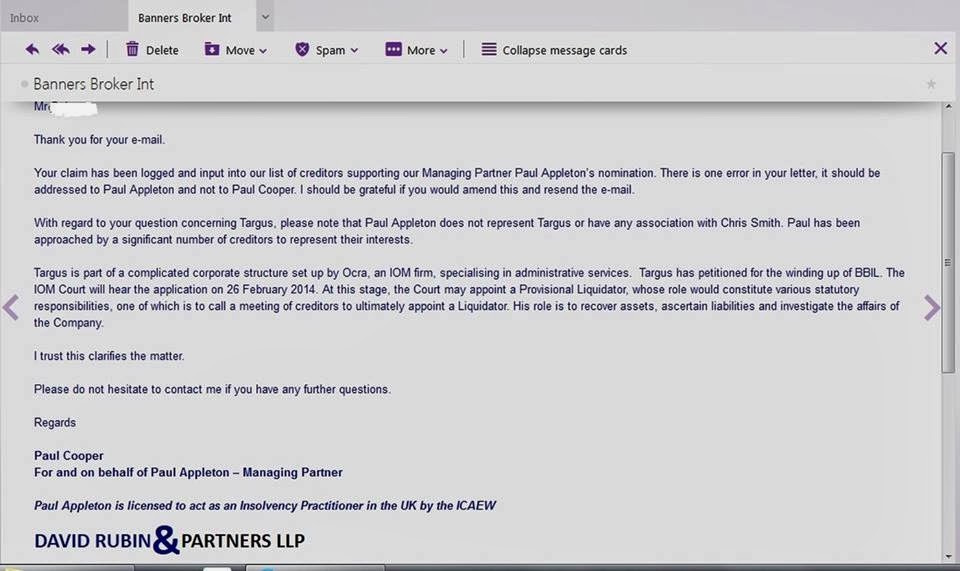Screenshot of an email on a light purple background from Banners Broker International. The header displays “Inbox” at the top, followed by “Banners Broker International” with a down arrow next to it. Navigation buttons include left and double left arrows, a right arrow, along with options to delete, move, mark as spam, view more options, collapse message cards, and an X button. 

The email begins with a repeated “Banners Broker International” header and a small dot next to it. The salutation “Mr.” is whited out for privacy. The email content reads:

"Thank you for your email. Your claim has been logged and input into our list of creditors supporting our managing partner Paul Appleton's nomination. There is one error in your letter; it should be addressed to Paul Appleton and not to Paul Cooper. I should be grateful if you would amend this and resend the email.

With regard to your question concerning Targus, please note that Paul Appleton does not represent Targus or have any association with Chris Smith. Paul has been approached by a significant number of creditors to represent their interest, and Targus is part of a complicated corporate structure set up by Okra, an IOM firm specializing in administrative services. Targus has petitioned for the winding up of BVIL. The IOM court will hear the application on 26th of February, 2014. At this stage, the court may appoint a provisional liquidator whose role would constitute various statutory responsibilities, one of which is to call a meeting of creditors to ultimately appoint a liquidator. His role is to recover assets, ascertain liabilities, and investigate the affairs of the company.

I trust this clarifies the matter. Please do not hesitate to contact me if you have any further questions. 

Regards, Paul Cooper For and on behalf of Paul Appleton, Managing Partner. Paul Appleton is licensed to act as an insolvency practitioner in the UK for the ICAEW. 

David Rubin and Partners LLP”

The message is flanked by navigation arrows, and the bottom section of the screenshot is gray, resembling a slide bar on the right side.